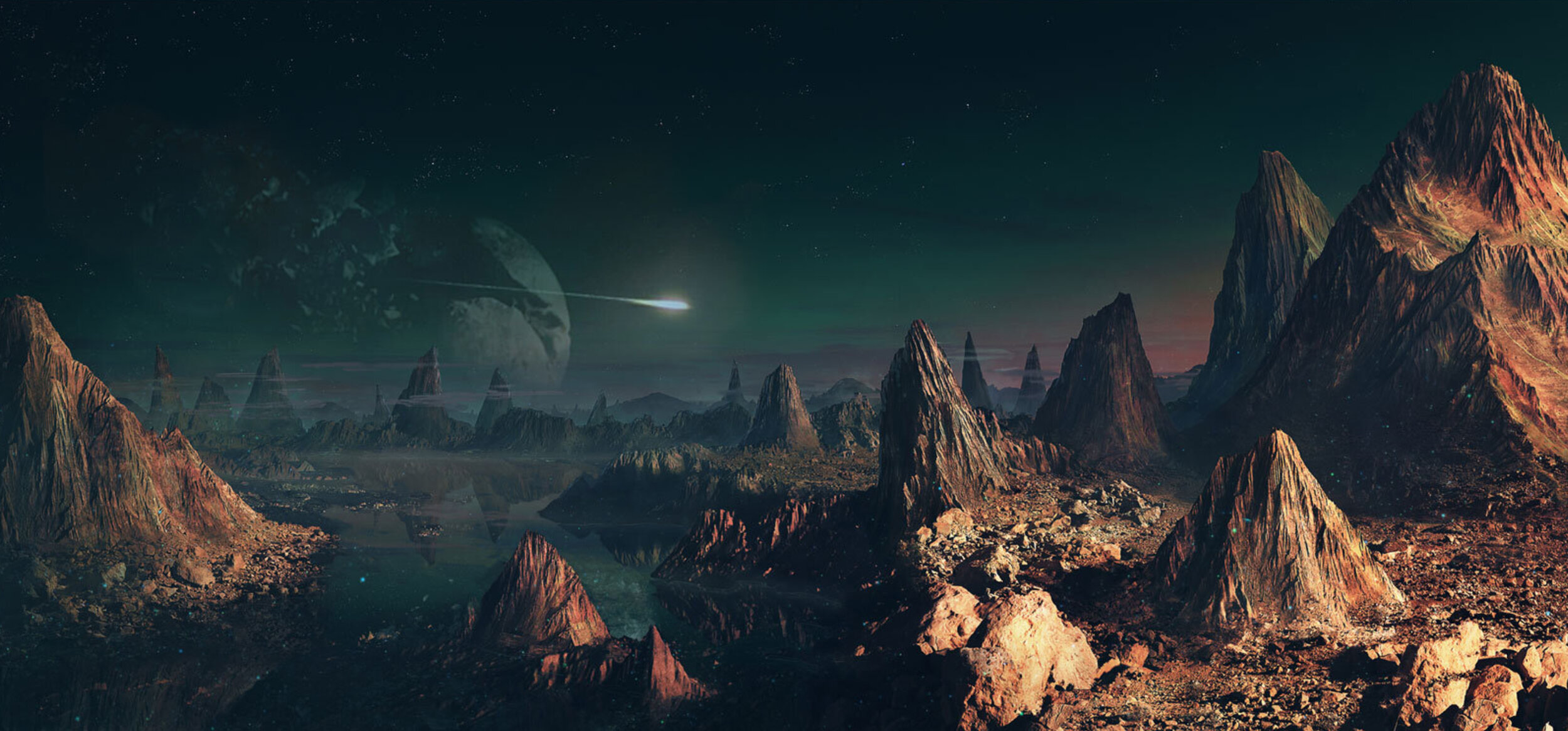This horizontally aligned rectangular digital art piece presents a striking, otherworldly landscape. The sky transitions from a solid black at the top into a dark gray with a faint purple tint near the middle, suggesting a planet's atmospheric gradient. Dominating this sky, a meteor streaks brightly across from the left to the center, emitting light. Behind it, in the far distance, looms a large, broken planetary body or moon, with jagged, fragmented edges.

In the background, sharply peaked, triangular rock structures emerge, shrouded partially by drifting clouds. These peaks are varied shades of gray, brown, and orange, contributing to the surreal ambiance of the scene. The foreground is filled with more triangular, jagged rock formations primarily on the right side, exhibiting a mix of medium and dark brown tones. The ground in this area is a rough blend of dirt and gravel.

Adding to the extraterrestrial feel, the lower left of the image features a body of water, bordered by additional craggy, pinkish-red and beige rock outcroppings. This detailed composition, from the alien sky to the rugged terrain, builds a vivid picture of a strange and intriguing extraterrestrial landscape.